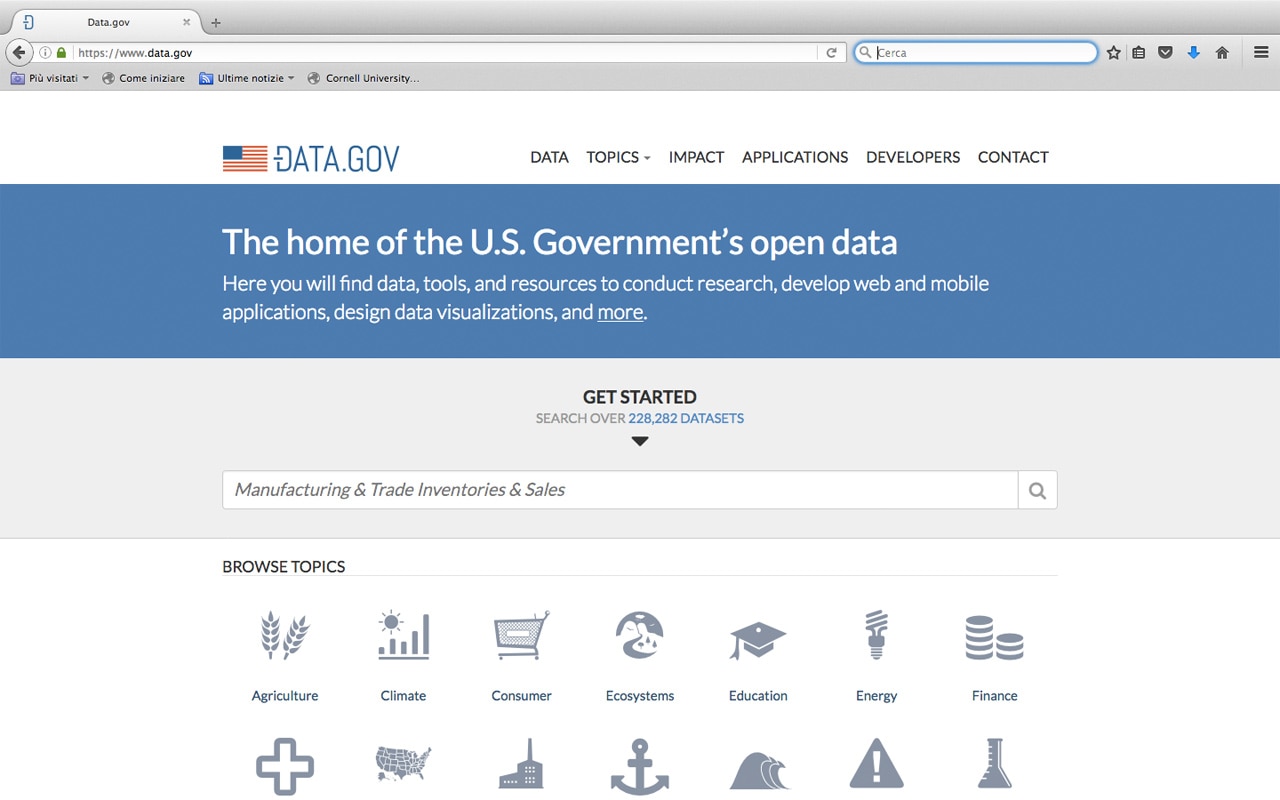This is a detailed screenshot of the official U.S. government website, data.gov. At the very top of the website, there's a white bar extending across the full width. In the top left corner, the government site logo, "data.gov," is prominently displayed in blue font, immediately to the right of a small American flag icon. Towards the right side of this white bar, the main navigation menu includes six options: 'Data', 'Topics' (which features a dropdown menu), 'Impact', 'Applications', 'Developers', and 'Contact'.

Beneath the white bar, a blue banner spans the width of the page. In large, bold white text, it declares, "The home of the U.S. government's open data." This banner further explains the purpose of the site with the text, "Here, you will find data, tools, and resources to conduct research, develop web and mobile applications, design data visualizations, and more." Notably, the word "more" is underlined, indicating it's a clickable link.

Below this blue banner, there is a gray section that invites users to "Get Started." In this area, a highlighted blue text line invites users to search "over 228,282 datasets," promising a vast repository of data available for public use.